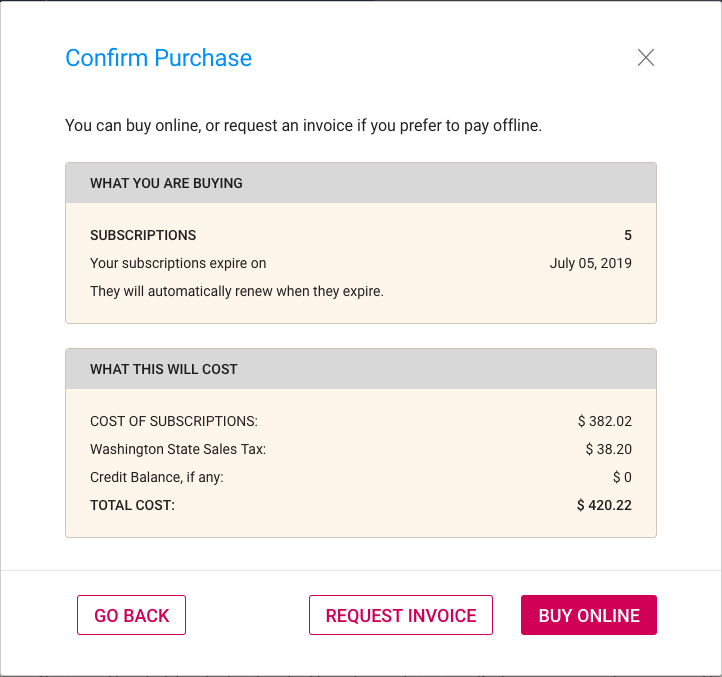A pop-up confirmation dialog appears on the computer screen, featuring a square box with an "X" in the top-right corner to close the window. The title at the top of the dialog reads "Confirm Purchase" in blue. Below this title, a message indicates the option to either buy online or request an invoice for offline payment.

The interface consists of two main sections within the pop-up:

1. **Subscription Details:**
   - The first section has a gray header with the text "What are you buying" in black font. Below this header, it lists the details of subscriptions noting, "Your subscriptions expire on July 5th, 2019. They will automatically renew when they expire."

2. **Cost Breakdown:**
   - The next section presents the pricing details within a similar gray header labeled "What will this cost."
   - **Cost of Subscriptions:** $382.02
   - **Washington State Tax:** $38.20
   - **Credit Balance (if any):** $0
   - **Total Cost:** $420.22

At the bottom of the pop-up, there are three buttons:
   - A white button with a red outline and text stating "Go Back."
   - A similarly styled button that says "Request Invoice."
   - A prominent red button with white text reading "Buy Online."

The pop-up uses a color scheme featuring blue, black, gray, tan, white, and red, and it appears to contain details about five subscriptions up for renewal.